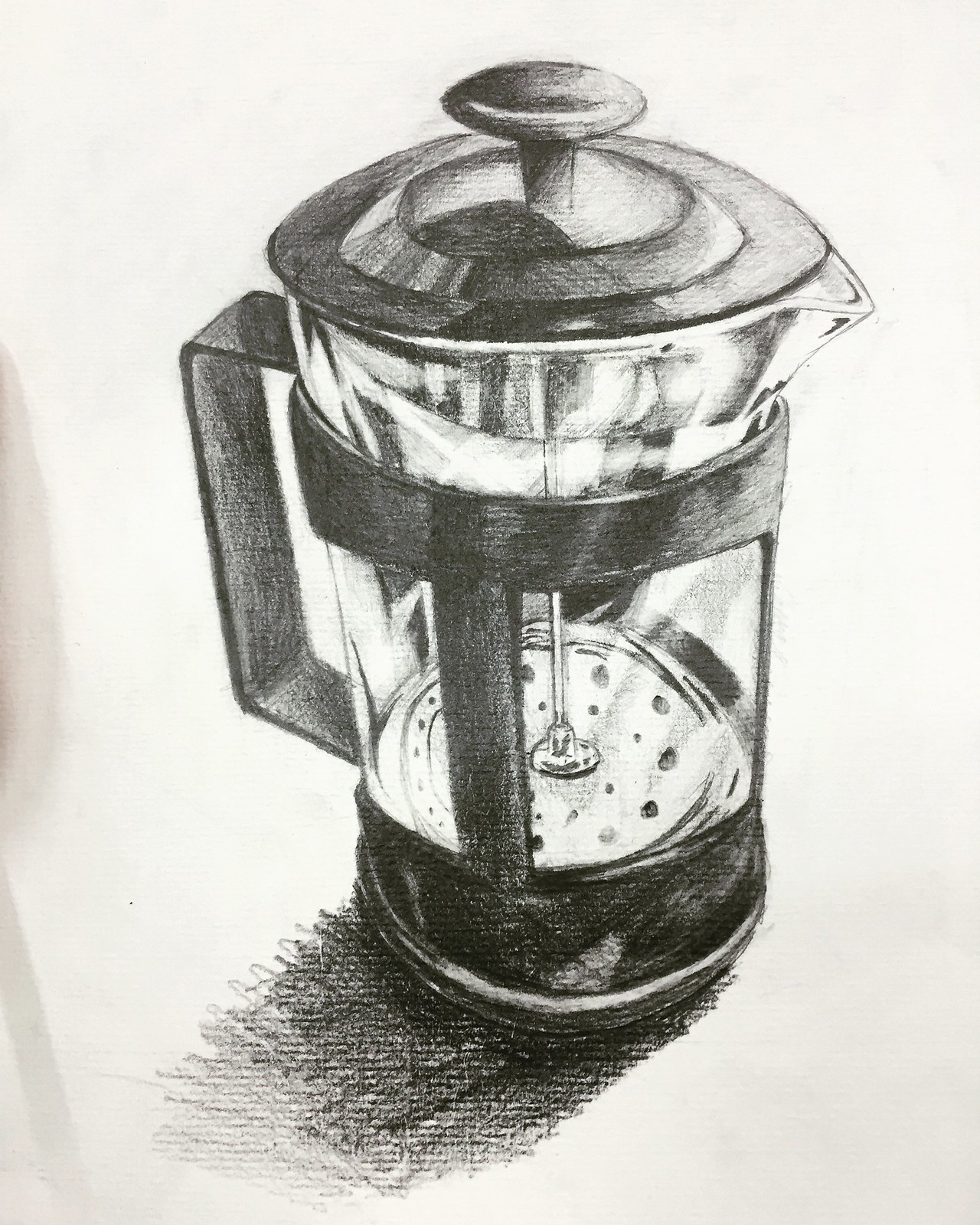This detailed pencil sketch, rendered in black and white on a blank white background, portrays a French-style coffee plunger pot, specifically a coffee press. The artist has meticulously used various shading techniques to create a three-dimensional effect throughout the sketch. The coffee press features a distinct round, flat knob at the top, leading down to the curvilinear structure of the pot. The lid is sketched in a dark black with slightly lighter shading towards the center. The body of the pot includes a visible stainless steel filter and clear glass section, allowing the internal components like the percolator and metal plunger plate to be seen. The pot is depicted as empty. On the side, there's a D-shaped handle extending from the pot, adding to the realistic quality of the drawing. Below, the object sits on a base that has been shaded darkly, hinting at the surface it is resting on. Overall, the artwork emphasizes the intricate details of the coffee plunger pot through skillful pencil work and deliberate contrast.